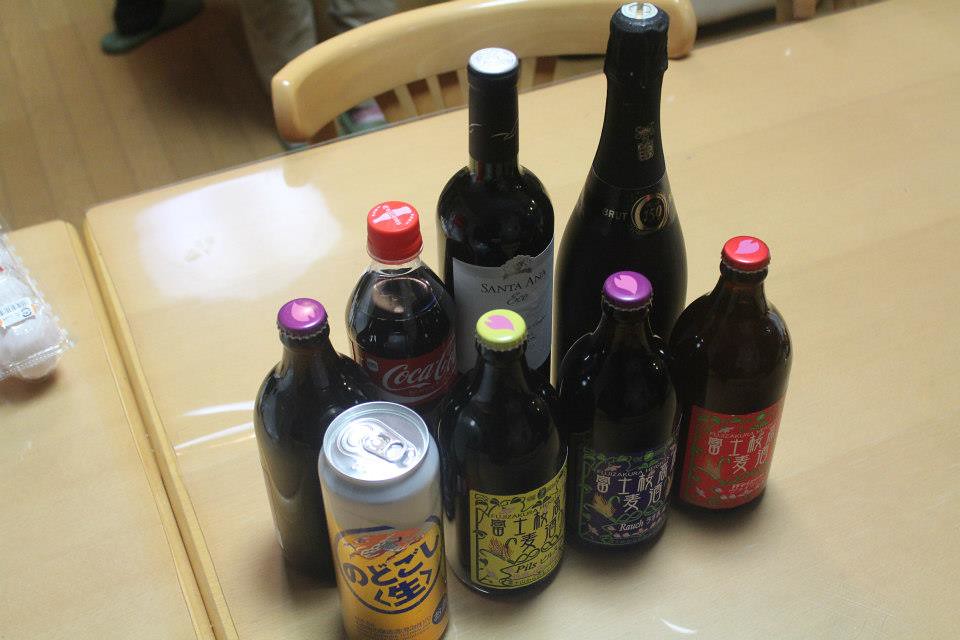The photograph depicts a yellow, shiny restaurant table with a matching chair pushed against it at the top of the image. On the table are eight containers: seven bottles and one can. The can is silver and gold with writing in another language. The seven bottles include two tall wine bottles with cork tops, a clear plastic Coca-Cola bottle with a red cap, and four shorter beer bottles with clamp-tight tops. The beer bottles each have different colored labels: one green, one blue, one red, and one yellow. The table rests on a wooden floor, adding a warm ambiance to the scene.